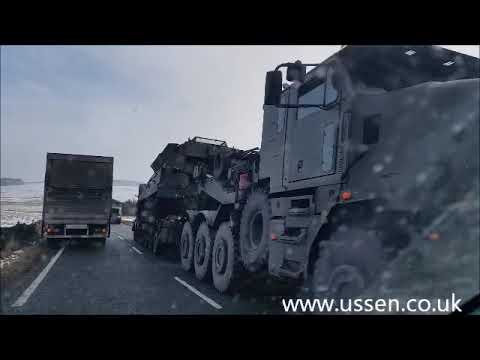This photograph captures a detailed scene of a narrow blacktop road on an overcast day with light rain. Prominently positioned in the image are large trucks, including a massive military truck hauling a large piece of machinery. This truck, with its massive tires, is primarily visible at a diagonal angle from the right side, extending towards the center of the image. Adjacent to this vehicle, the back end of a filthy black box truck is seen to the left, partially on the road shoulder to allow passage. The road itself is detailed with a solid white line on the left edge and a white dotted line running through its center, extending into the distance. On the left side of the road, there is a bunch of weeds and mud, while the background features a body of water under a sky filled with white clouds. The web address "www.ussen.co.uk" is displayed in white letters in the bottom right corner of the image. Additionally, the photograph is bordered by two horizontal black strips at the top and bottom.